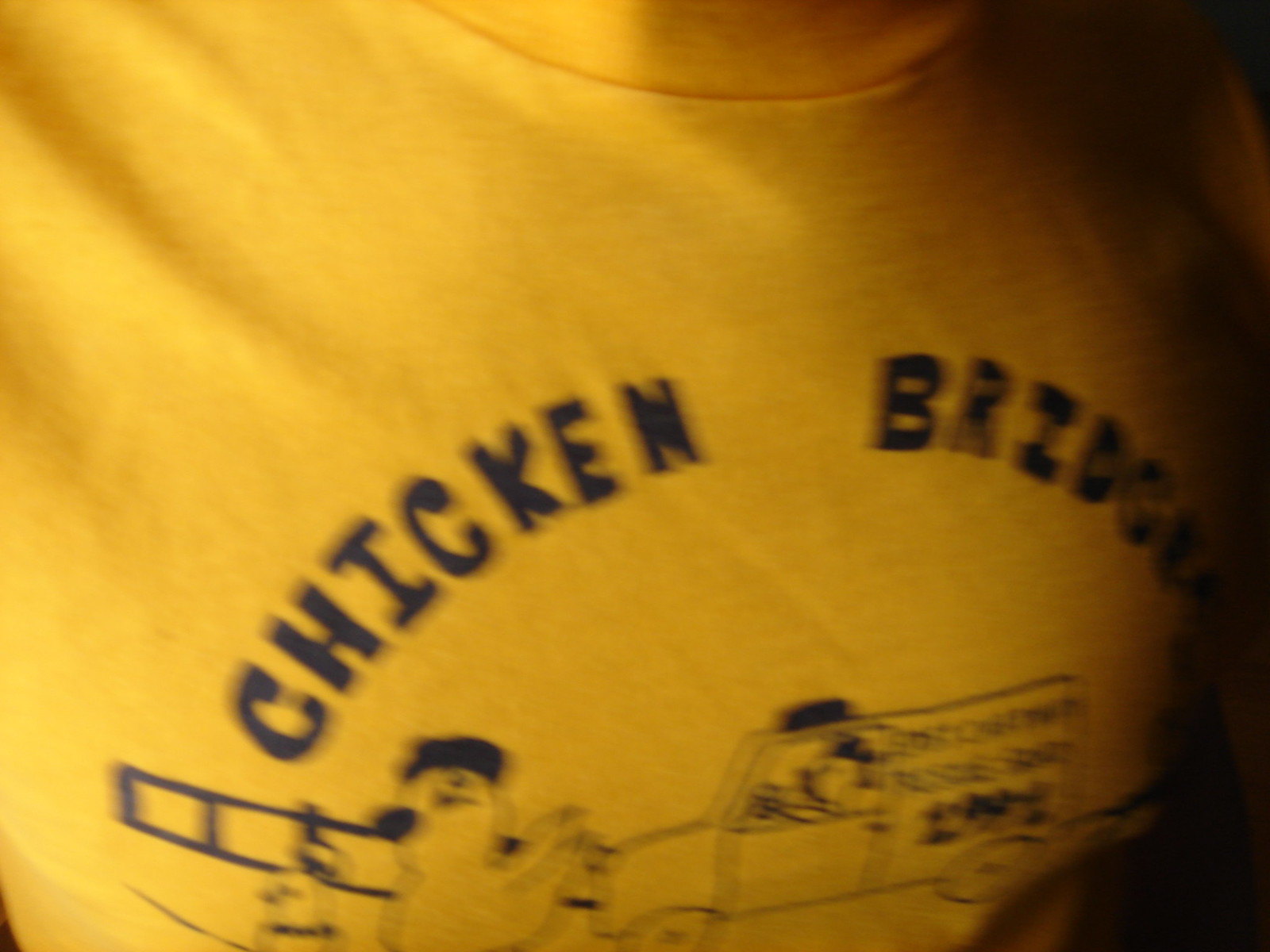The image showcases the front of a person's mustard-yellow t-shirt, visible from their neck to their chest. The shirt features bold, black capital letters spelling "CHICKEN" across the chest. Below this, only the first four letters "B-R-I-D" of another word, presumably "BRIDGE," are visible, as the remaining part of the word is obscured.

Beneath the text is a detailed black graphic. This graphic depicts a fence with several chickens in front of it. Behind the fence, there is a truck with a siren on top, suggesting it might be an emergency vehicle or a delivery van. Notably, the truck appears to be driven by a chicken. Parts of the writing on the side of the van are blurry and hard to decipher, but the number "1991" is discernible. The overall impression is that the t-shirt advertises a chicken-related business or shop, potentially named "Chicken Bridge," though the exact bottom part of the graphic remains out of focus in the image.